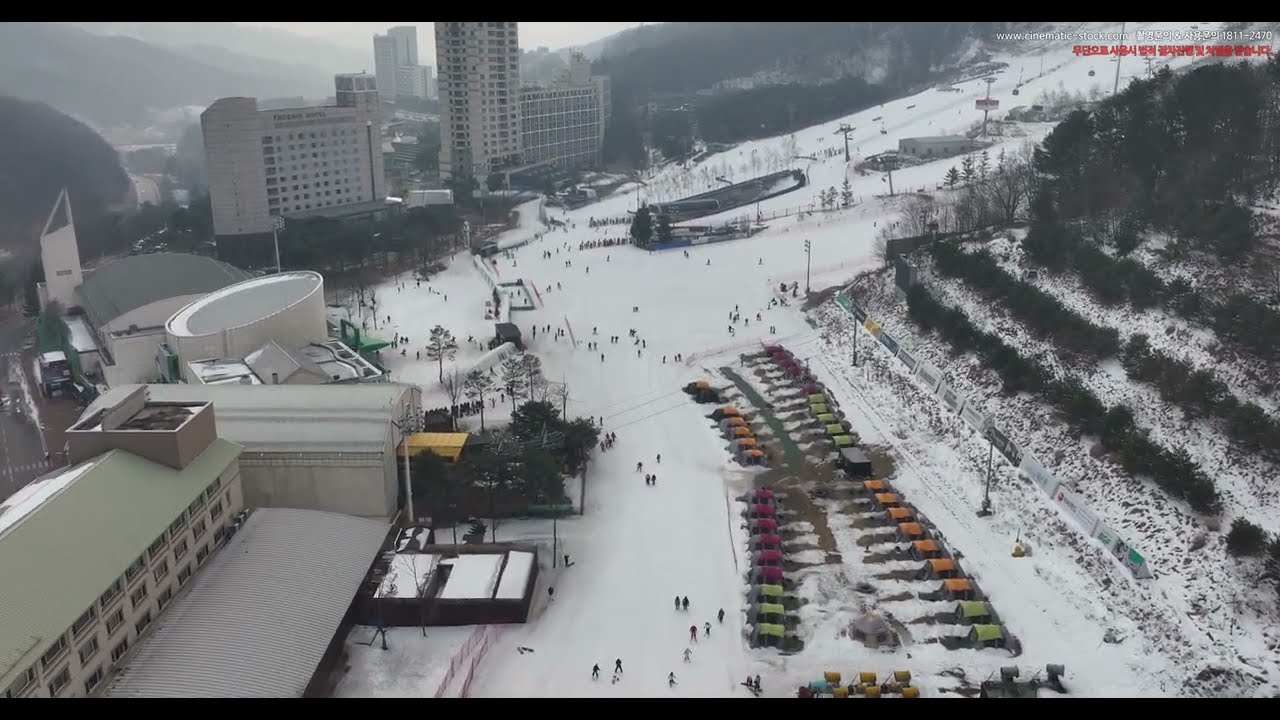The image captures an expansive, snowy landscape in what appears to be an Asian metropolitan city. The setting is reminiscent of a ski resort, with a multitude of large buildings, identified as possible condos or hotels, scattered throughout the scene. To the left side of the image, prominent structures such as the "Phoenix Hotel" can be observed, indicating a well-developed area amidst the wintry conditions. The foreground features numerous people walking and skiing on the snow-covered terrain, with clusters of skiers descending a nearby slope. Hills and obscured details by fog are visible in the background, enhancing the scenic depth of the image. Various colored capsules are positioned off to the right, adding a splash of color to the predominantly white and gray snowy expanse. Notable colors in the image include white, light green, red, orange, yellow, green, gray, and black, offering a vivid and dynamic visual palette. The scene is blanketed with snow, complemented by sparse patches of grass, and the activity of numerous skiers centralizes the snowy action. There are no legible texts within the main frame, but references to Asian scripts and website details from www.cinematic-dot.com suggest an origin in northern Japan or China. The overall image, captured during daylight, provides a dynamic, wintry snapshot of a bustling, outdoor, metropolis imbued with the serene beauty of a snowy day.